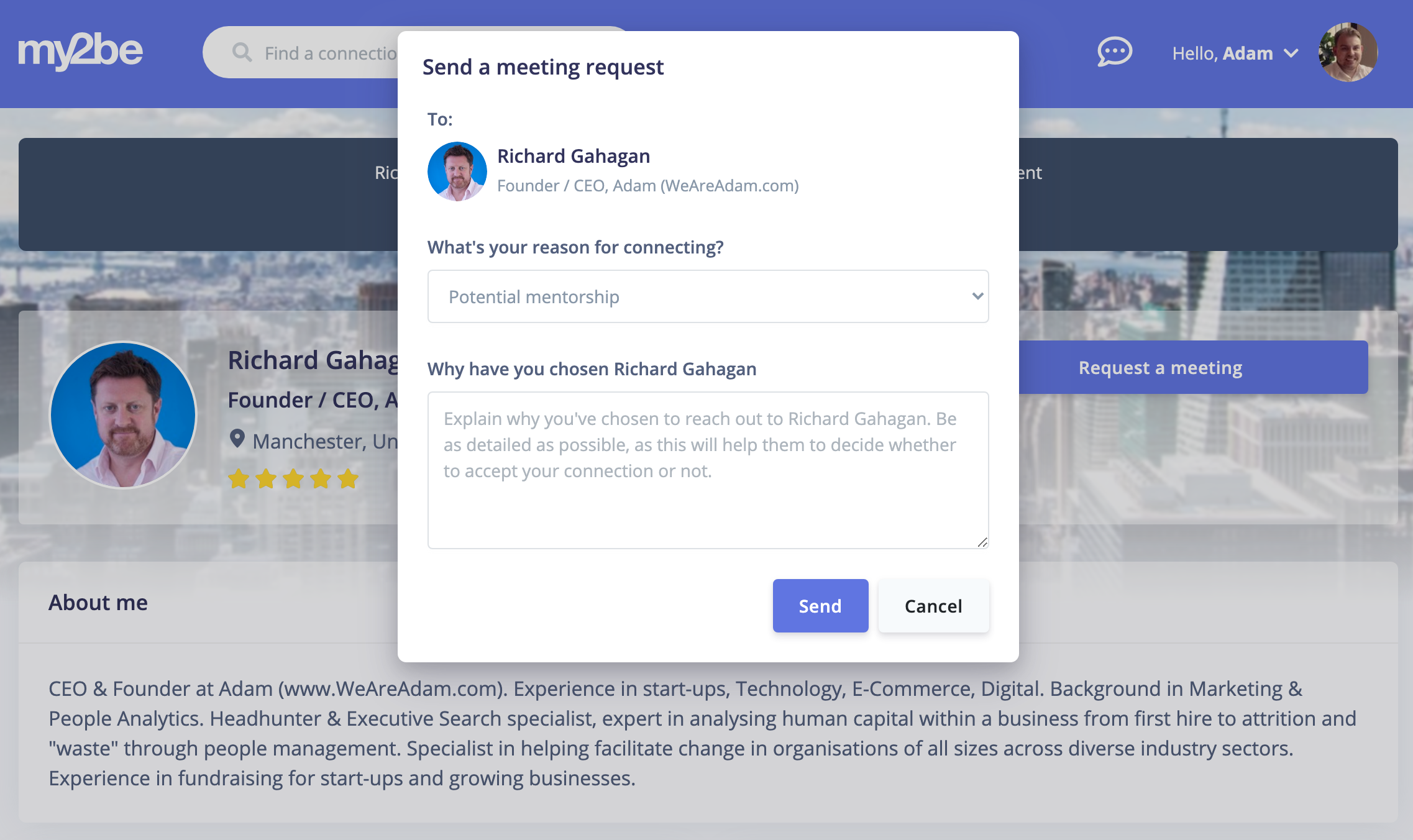This image is a screen capture from a web-based platform called "my2b". The interface prominently features a navigation strip at the top with a search bar and a small speech bubble that greets the user with "Hello Adam." Next to this greeting is a dropdown menu and a circular icon showcasing Adam's profile picture, which partially obscures a section of the webpage.

The main content of the page is a form for sending a meeting request to Richard Gahagan, who is identified as the Founder and CEO. The interface asks Adam to provide a reason for connecting, selectable from a dropdown menu that currently shows "Potential Mentorship." Beneath this, there is a prompt titled "Why have you chosen Richard Gahagan?" accompanied by a text box where Adam is instructed to explain his reasons for reaching out in detail, to aid Richard in deciding whether to accept the connection request.

The form is accompanied by "Send" and "Cancel" buttons. In the background, partially obscured by the white overlay of the form, is Richard Gahagan's profile, identifiable by his picture and partially visible name. To the right, there is a "Request a Meeting" button, and the background image behind Richard's profile appears to be a cityscape. At the lower portion of the screen, Richard's "About Me" section provides additional information about his identity and business endeavors.